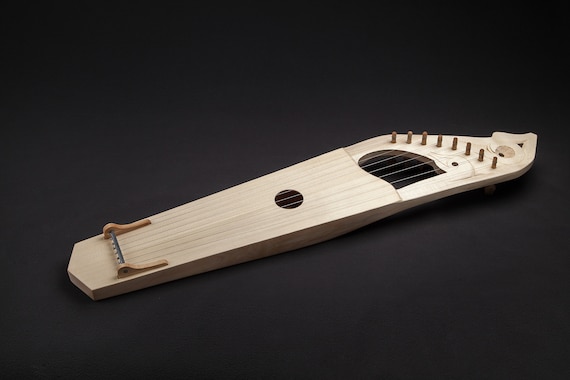This is a photograph of a unique, light-colored wooden string instrument resembling the Japanese koto. The instrument, which lies flat on a dark gray and black background, features a long, rectangular body with geometric precision. It is equipped with nine strings, each string stretching from a bar at the bottom end to nine pegs arranged in a curved, equally spaced manner at the top end, providing tunable adjustments. Near the bottom left of the instrument, there is a circular hole, while towards the top, a smaller, backward D-shaped cutout is present, potentially for a handhold. The top end also showcases an elegant design, possibly a bird's head above the smaller hole and a tip with a wavy lotus-like finish. The instrument, intriguingly different from Western stringed instruments, bears a distinct aesthetic and functional form.